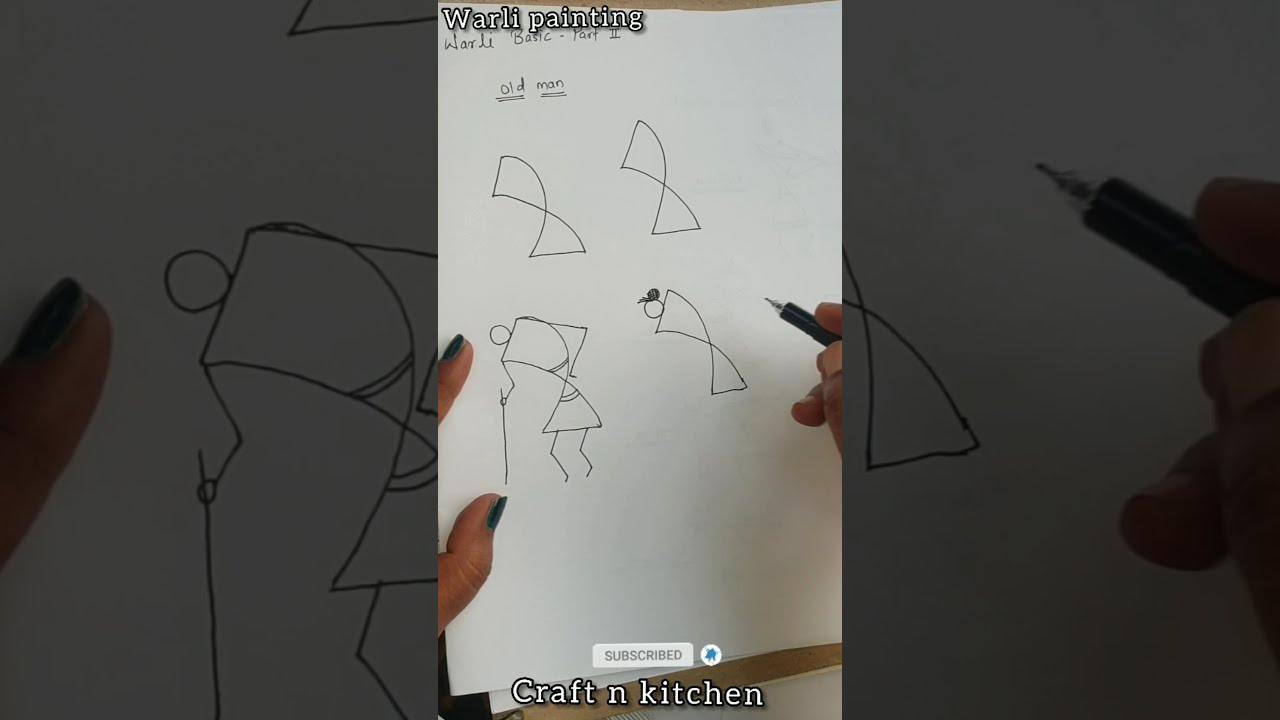The image is a vertical cell phone photo centered on a piece of paper with a zoomed-in and faded version of the same photo as the background. The paper shows four different sketches arranged in a rectangular grid. At the top of the sketches, the handwritten text "Old Man" is prominently displayed, with each word double underlined. The top two sketches are curved triangular geometrical shapes with two intersecting lines. The bottom two sketches evolve these shapes into simplistic stick figures representing an old man bent over holding a cane. Hands, seen on the left and right sides, are actively sketching with a pen or mechanical pencil, suggesting a first-person view. Along the top of the image, the text "Worli Painting" is written, while "Craft in Kitchen" is printed at the bottom. The image features colors such as white, black, brown, blue, and dark green, resembling a screenshot from a mobile device, possibly intended for social media.